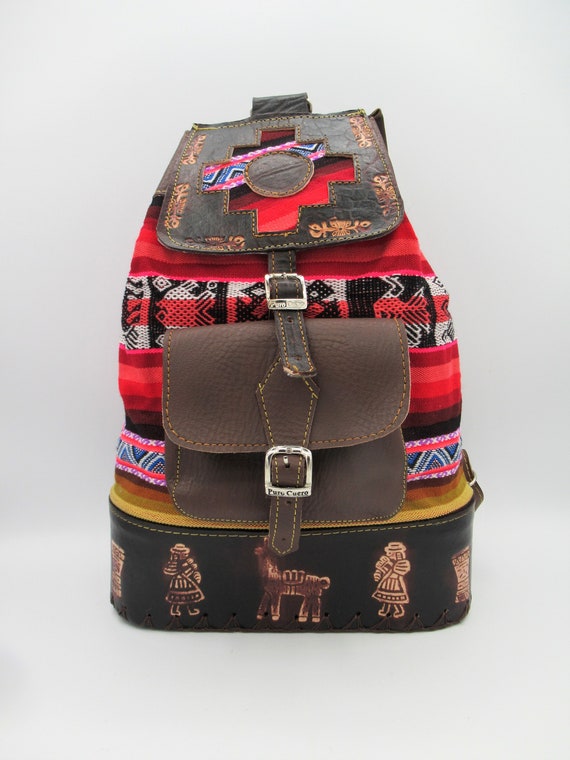This image captures a vividly colorful backpack with a Mesoamerican-inspired design. The shot is taken from the bottom of the backpack, which is laid flat on a table. The base of the bag is crafted from black leather and is adorned with intricate stamped images depicting llamas and women in traditional dresses and hats, highlighted in yellow details. Moving upwards, a section of the backpack features a vibrant woven fabric with alternating patterns of pink stripes and blue and black triangles, displaying a dynamic back-and-forth design. Above this, there is a series of red stripes with varying shades, ranging from dark burgundy to lighter reds, interspersed with black banding and faint red stripes incorporated into black and white symbols.

The middle section of the backpack continues with a rich combination of hues, showing darker and lighter red stripes mixed with deeper burgundy tones against black fabric. At the top of the backpack, a dark brown leather flap, stamped with designs, folds over to close the bag. This flap features a leather strap bearing the same pink and blue triangular pattern, secured by a silver buckle. Additionally, attached to the front of the flap is a smaller purse-like pocket, also constructed from dark brown leather with a silver clasp, further enhancing the texture and functionality of the backpack. The main body of the bag is predominantly constructed from red canvas, accentuated with various shapes that resemble fish, completing the intricate and culturally rich design.